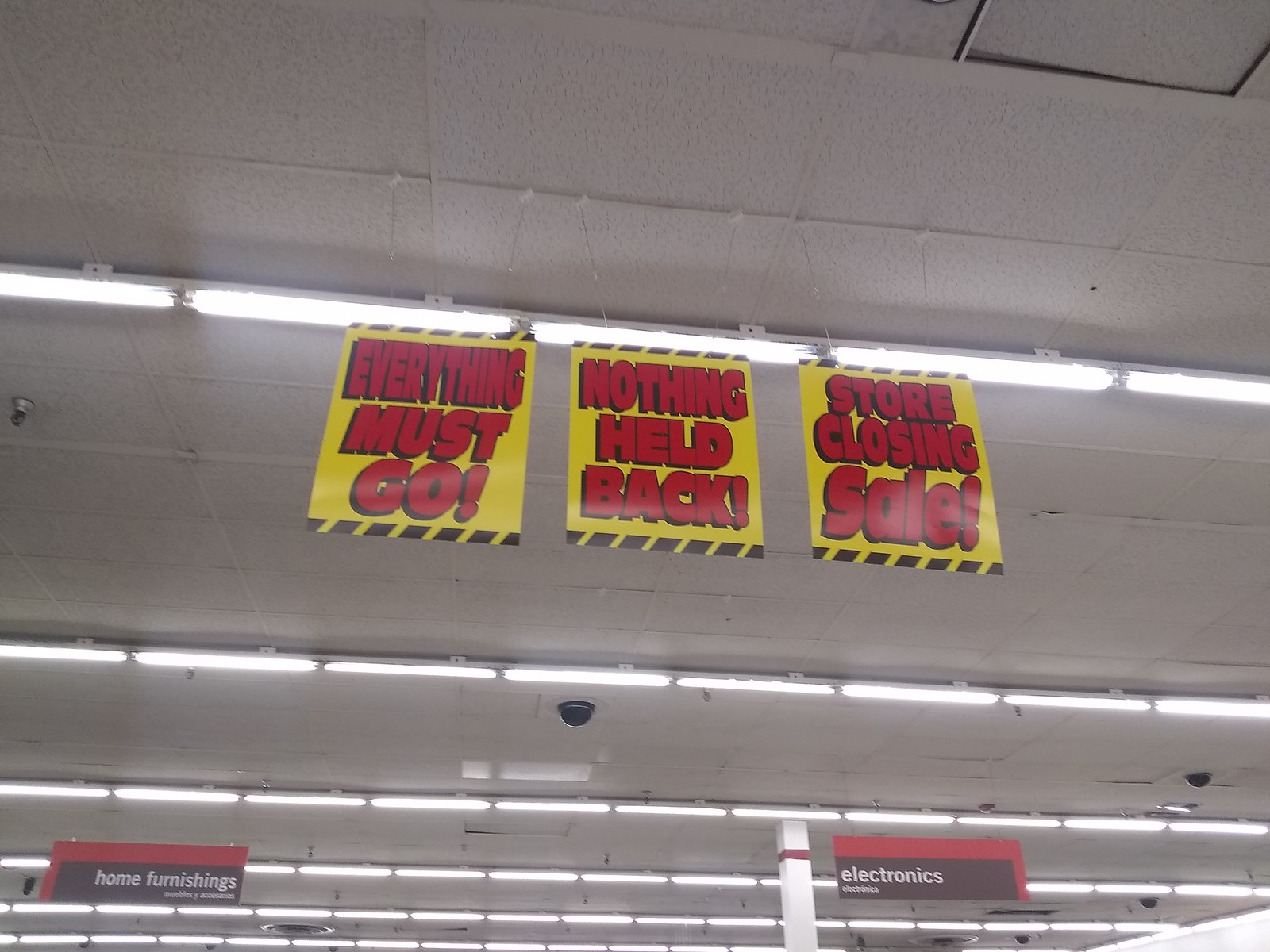This is an image looking up at the ceiling in a large department store. The ceiling features long rows of fluorescent tube lights with equal spacing, casting an even illumination across the white, tiled expanse. Sprinkled among the tiles are black glass domes, presumably housing security cameras. Dominating the scene are three large, square banners hanging from the ceiling. Each banner has a yellow background with alternating black and yellow dashes at the top and bottom edges. The left banner boldly declares "Everything Must Go" in giant red letters with a black background. The middle banner announces "Nothing Held Back" in red writing, also on a black background. The rightmost banner reads "Store Closing Sale" in large red letters outlined in black. Additionally, in the bottom left corner of the image, there's a black sign with a red border that says "Home Furnishings" in white text. On the bottom right, another similar sign reads "Electronics." The ceiling tiles feature a pattern of small dots, adding texture to the store's interior.